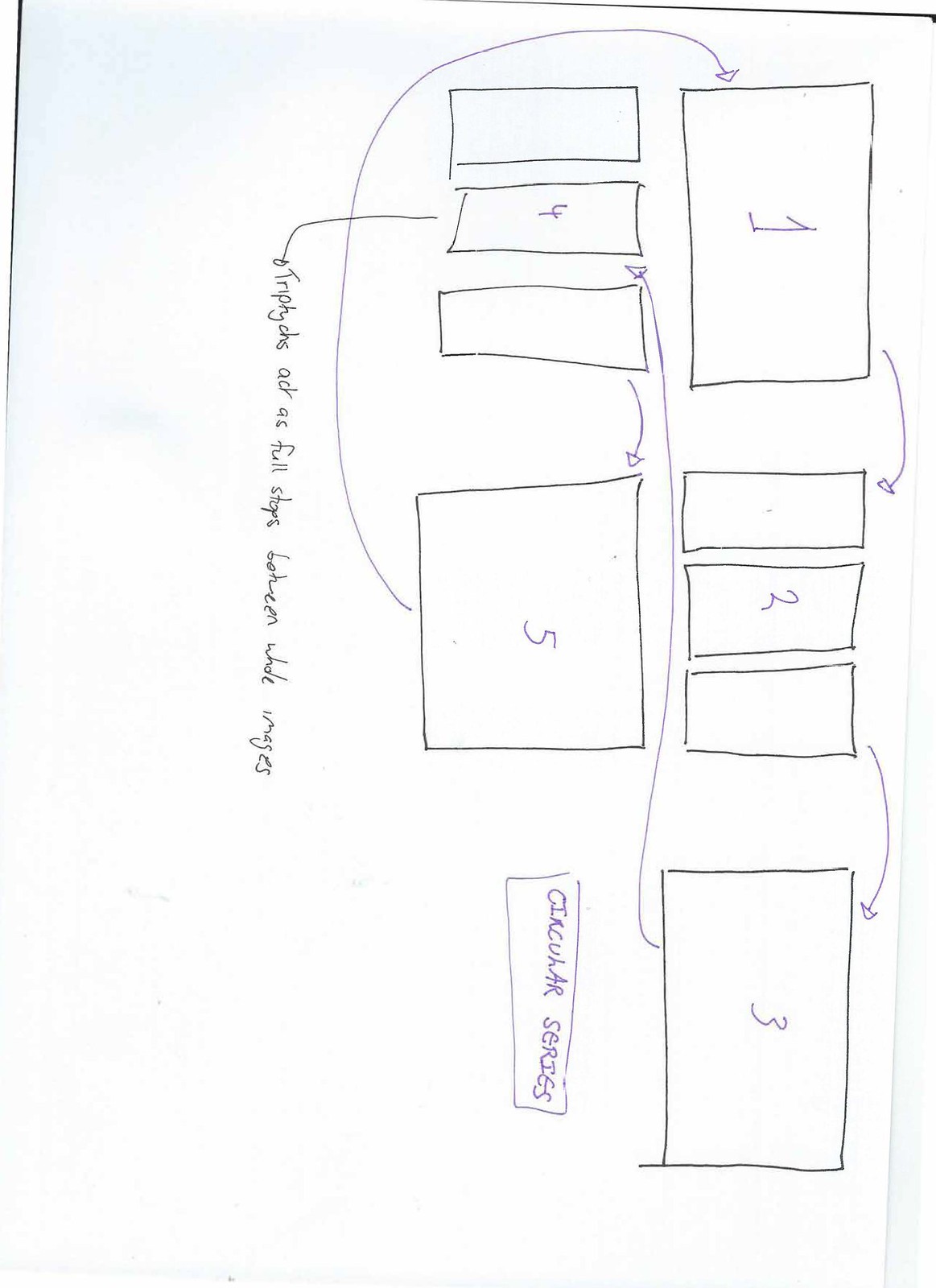A hand-drawn vertical diagram, incorrectly oriented to the left, is displayed on white paper. The diagram consists of several rectangular boxes connected by arrows, all meticulously drawn in black ink. 

The diagram begins with a single box labeled "1," from which an arrow points upward to a cluster of three rectangular boxes labeled "2." The boxes in this cluster are horizontally aligned.

To the right of the "2" cluster, a larger solitary box is marked with the number "3." From here, an arrow leads downwards to another trio of boxes, this time vertically aligned and labeled "4." Below the "4" boxes, an arrow points downward with the text, "Trifix act as full stops between whole images."

Continuing, another arrow connects to a single box labeled "5," which then loops back around to the box labeled "1," forming a circular series. The arrows and numbers are drawn in a bluish-purple ink, contrasting against the simplicity of the black-inked boxes and the stark white paper background.